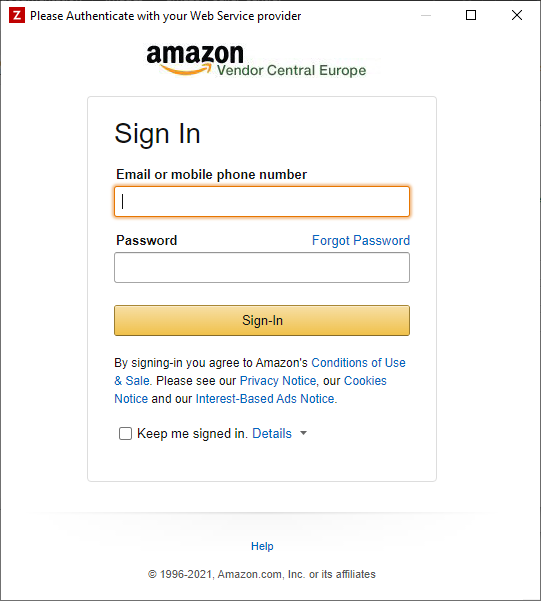This image depicts a detailed screenshot of an authentication window for Amazon Vendor Central Europe. The window, which appears to be a pop-up, is titled "Please authenticate with your web service provider," with a red Z-like symbol to the left of this text. On the top-right corner of the window, there are options to minimize, expand, or close the window.

At the center of the window is the Amazon Vendor Central Europe logo, featuring the classic Amazon black text with an orange arrow below and the text "Vendor Central Europe" in green underneath it. The authentication form includes a section titled "Sign in," prompting the user to enter an "Email or mobile phone number" in a highlighted text box with an active cursor. Following this, there is a "Password" field and a blue "Forgot password" link to the right.

Beneath the password field, there's an orange sign-in button for users to submit their login information. The text below the sign-in button states, "By signing in, you agree to Amazon's Conditions of Use and Sale. Please see our Privacy Notice, our Cookies Notice, and our Interest-Based Ads Notice." A checkbox labeled "Keep me signed in" with an accompanying "Details" arrow is positioned below this disclaimer. At the bottom, a blue hyperlink labeled "Help" provides additional assistance, and the window concludes with the copyright notice: "© 1996-2021, Amazon.com, Inc. or its affiliates."